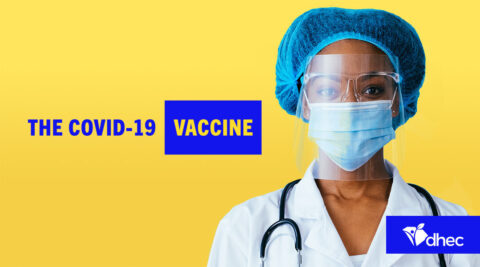This photograph features a female healthcare professional, presumably a nurse, positioned on the right side of the frame in a close-up shot that captures her face, head, and upper chest. She is clad in a white medical coat, accessorized with a stethoscope draped over her shoulders—the earpiece on her right side and the chest piece on her left. The nurse is equipped with several pieces of personal protective equipment, including a blue hairnet, a face mask, a transparent face shield, and a pair of glasses. She gazes directly into the camera with a serious and composed expression. To her right, on the left side of the image, the words "COVID-19 Vaccine" are prominently displayed, while the bottom right corner features the acronym "DHEC," indicating the involvement of the Department of Health and Environmental Control.